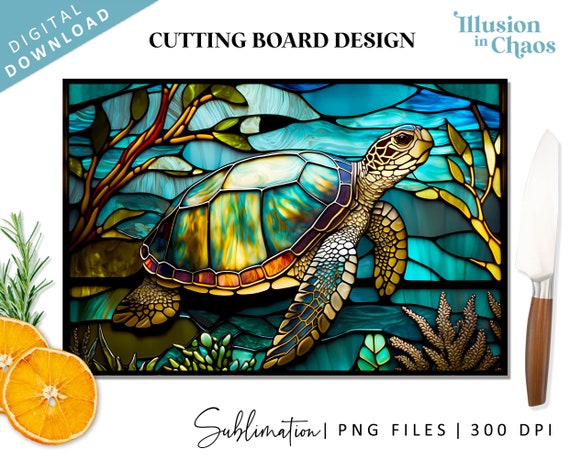This is an advertisement for a digital download featured on a white background. Central to the image is an ornate stained glass-style art piece showcasing a sea turtle with a variegated shell featuring hues of yellow, blue, and green, and olive-colored scales on its body. Surrounding the sea turtle are detailed coral and underwater plant life, enhancing the marine theme, while multiple shades of blue waves in the background evoke a sense of being underwater. The top of the image displays a black header that reads "Cutting Board Design," flanked by "Digital Download" in a blue triangle on the upper left corner and "Illusion in Chaos" in matching blue font on the upper right corner. The bottom text, also in black, indicates "Sublimation PNG files 300 DPI." On the lower left corner, two slices of orange and a sprig of rosemary slightly cover the cutting board, adding a touch of culinary context. To the right, parallel to the cutting board, is a knife with a wooden handle and a light silver blade, reinforcing the practical aspect of the design.